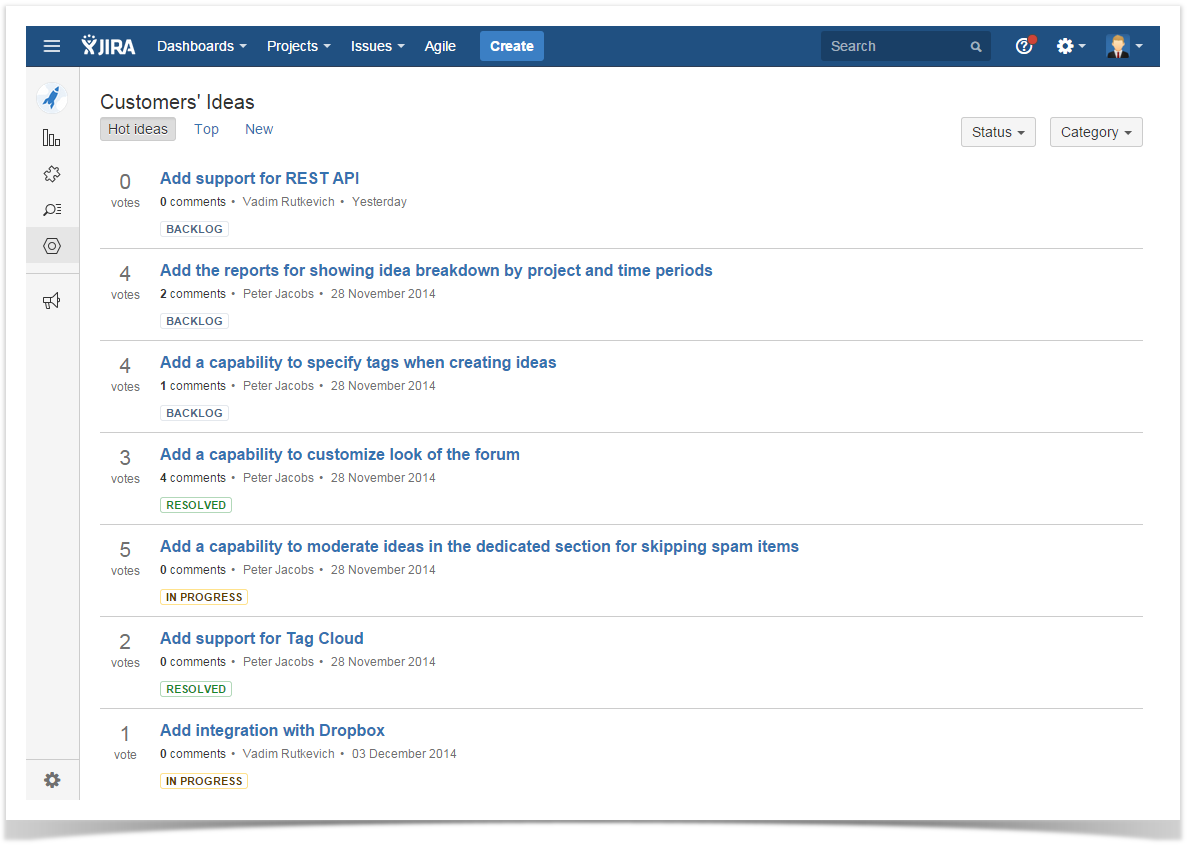This image is a screenshot of a website displayed in landscape mode. The interface is dominated by a dark blue top bar that houses several key elements. In the upper left-hand corner, there is a three-line icon for additional options, followed by a logo that resembles an intertwined X, accompanied by the text "JIRA." Next to the logo are several drop-down menus labeled "Dashboards," "Projects," "Issues," and "Agile." A blue "Create" button is positioned prominently, and the rightmost section of the bar includes a search bar, a help icon represented by a question mark in a circle, a notification bell, a settings gear, and an avatar of a light-skinned male in a suit and tie, which also has a drop-down menu.

The main part of the screenshot is predominantly white, except for a left sidebar featuring icons: a rocket, a graph, a puzzle piece, a search icon, and a highlighted gear, with a "Announcements" label above. This gear icon suggests that the current page is related to settings or configurations.

In the main section, the second column is topped with a header that reads "Customers Ideas," accompanied by a series of buttons: a gray one labeled "Hot Ideas," and a prominently colored blue one labeled "Top." Adjacent to these are additional options like "New," as well as drop-down menus for filtering by "Status" and "Category."

Below these controls are seven rows of content, each depicting specific ideas with corresponding vote counts. The rows are detailed as follows:
1. Zero votes - "Add support for REST API"
2. Four votes - "Add the reports for showing idea breakdown by project and time period"
3. Four votes - "Add a capability to specify tags when creating ideas"
4. Three votes - "Add a capability to customize look of the forum"
5. Five votes - "Add a capability to motivate ideas in the dedicated section for skipping spam items"
6. Two votes - "Add support for tag cloud"
7. One vote - "Add intent creation with Dropbox"

At the bottom of each row are small buttons indicating the status of each idea: "Backlog," "Resolved" (in green), and "In Progress" (in brown).

This detailed layout suggests that the screenshot is from a project management or issue-tracking platform, specifically presenting an interface for managing customer feedback or ideas.